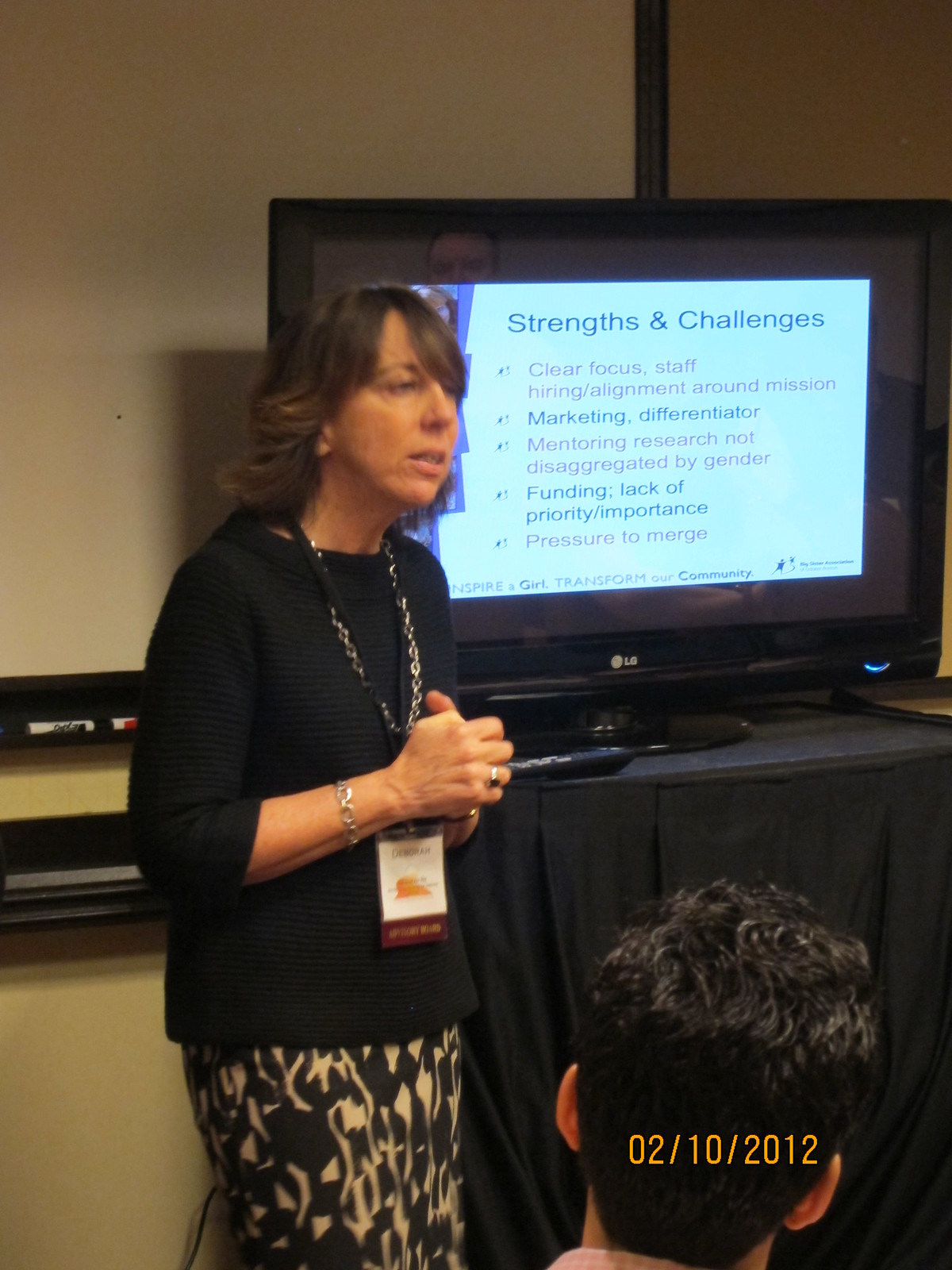In a color photograph taken on February 10, 2012, a woman named Deborah is presenting a seminar. She stands on the left side of the portrait-oriented image, distinguished by her medium-length dark brown hair, a silver necklace, and a black top paired with a black and gold patterned skirt. Accessories include a bracelet on her right wrist and a ring on her right ring finger. Around her neck, she wears a black lanyard with a white name tag. Behind her, a monitor displays the heading "Strengths and Challenges" in blue text, with bullet points such as "Clear Focus," "Staff Hiring," and "Alignment Around Mission," among others, listed below in red and black text. The monitor rests on a black table draped with a black cloth. In the bottom right corner of the image, the back of an audience member's head with black hair is visible, emphasizing that Deborah is addressing an audience. The date stamp, "2-10-2012," appears in gold at the bottom right. The overall style of the photograph is Photographic Representationalism Realism.